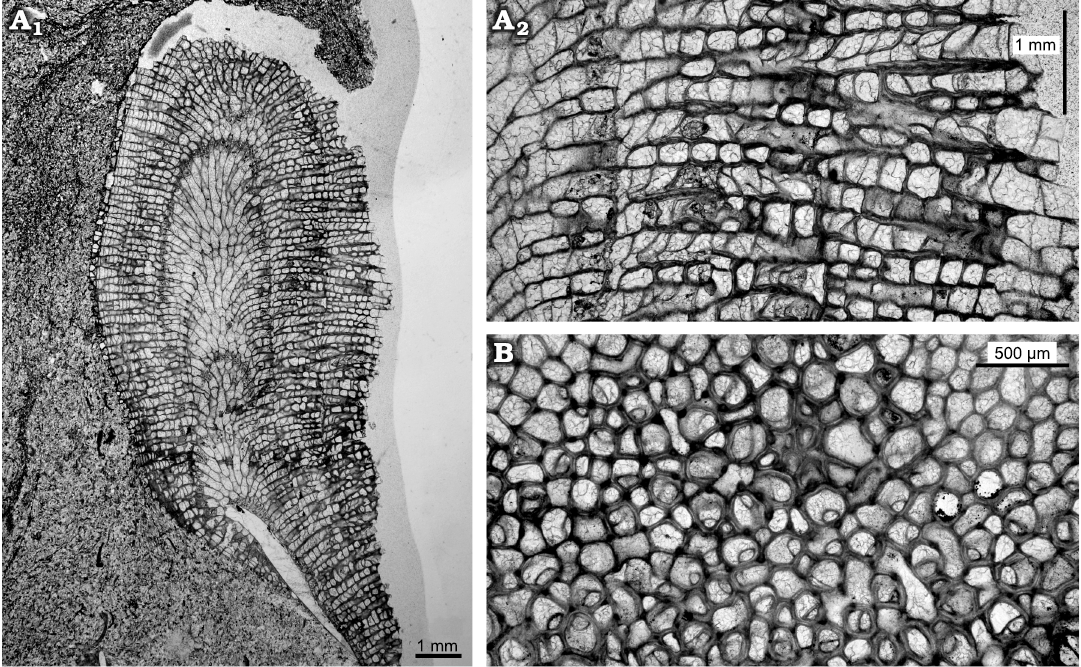The image is a three-part black and white composite photograph labeled as A1, A2, and B, arranged in a grid. A1 is a vertical photo on the left, while A2 and B are stacked on top of each other on the right. A1, with a scale of 1mm, appears to show a magnified cell structure or perhaps an x-ray image, resembling tree bark or a microscopic view of cellular formations, with numerous cell walls visible. A2, which is positioned above B, displays a closer view at a scale of 1mm, detailing these structures further with distinct dark lines separating lighter, whitish-gray vascular-like regions. B, located beneath A2 and showing an even more magnified view with a scale of 500um, presents roundish, tightly packed pebble-like forms, which might be further magnified cells or another layer of the same biological sample. The precise nature of the images—whether they depict a medical condition, plant cells, or another sample—remains unclear but their detailed structural presentation indicates a significant magnification.